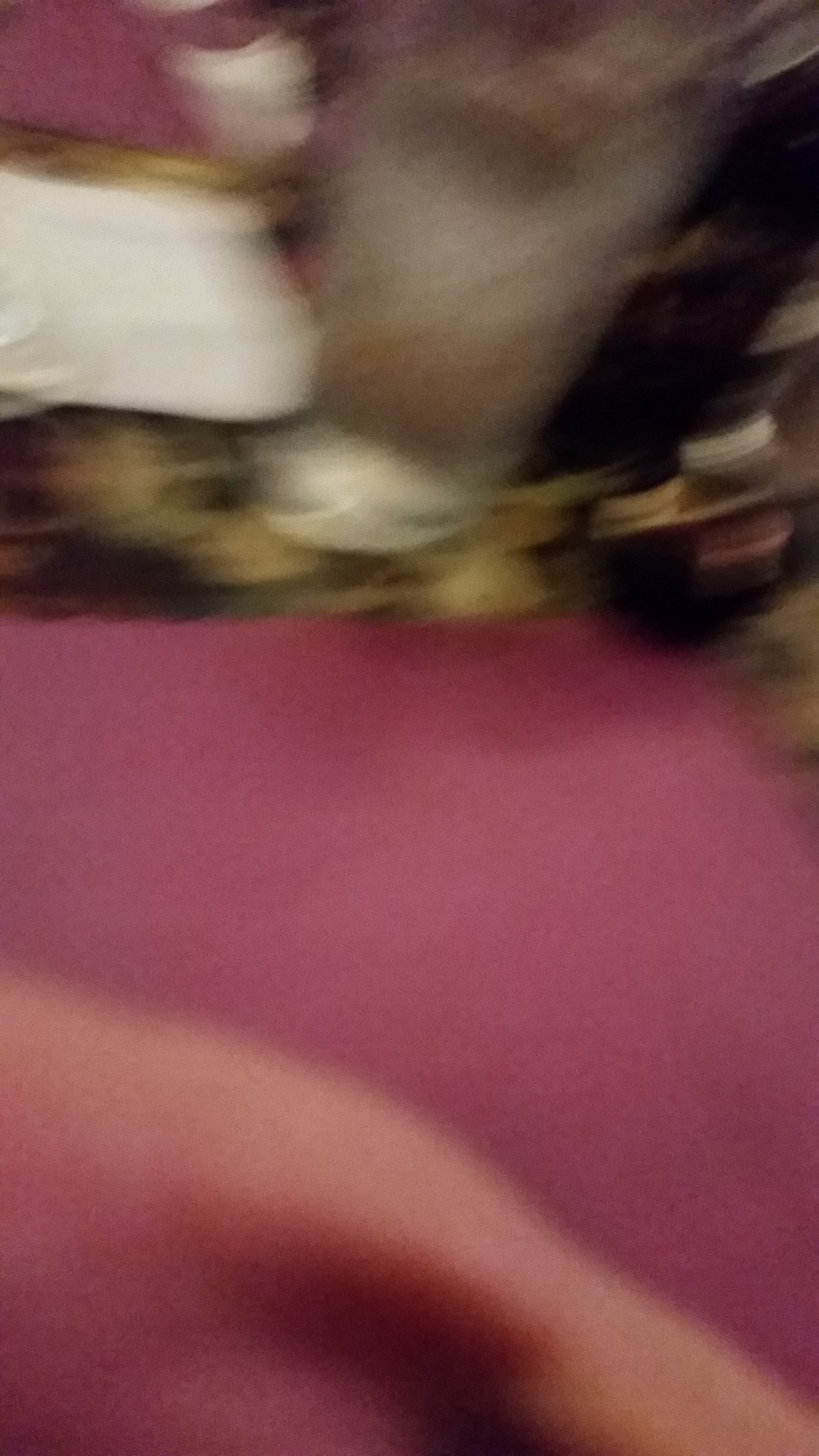The image is a blurred, indistinct composition where only colors and vague shapes are observable. Central to the image appears to be a floor showcasing a floral design. Emerging from the bottom and extending beyond the center is a pinkish object, which has a section on the left side that transitions to a lighter, skin-tone hue. Toward the top of the image, there are indistinct objects that range in color from white to gray. The overall effect is a blend of soft tones and forms, creating an abstract, almost dreamlike visual.